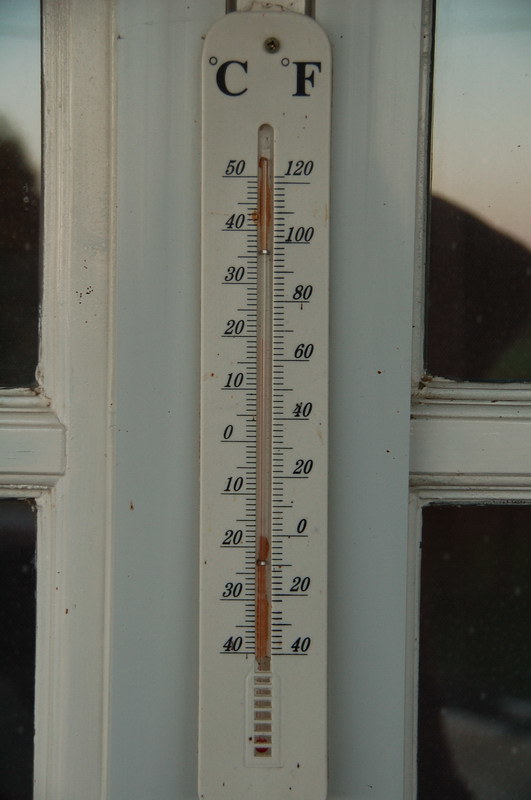In this image, we see an outdoor thermometer affixed to a vertical piece of white-painted wood trim beside a window. The window is divided into four panes of glass by a central bar, with two panes on each side. The thermometer, which is slightly faded to an off-white color, is secured in place by a screw at its top. It features large black letters "C" for Celsius and "F" for Fahrenheit at the top. The red mercury level is low, indicating a temperature of around 0 degrees Fahrenheit or 20 degrees Celsius. The Celsius scale ranges from -40 to 50 degrees, while the Fahrenheit scale goes from -40 to 120 degrees, with small black tick marks for precision. Below the mercury-filled glass tube, there is a vent-like section with seven small cut-out squares that are a brighter off-white, contrasting with the rest of the thermometer.